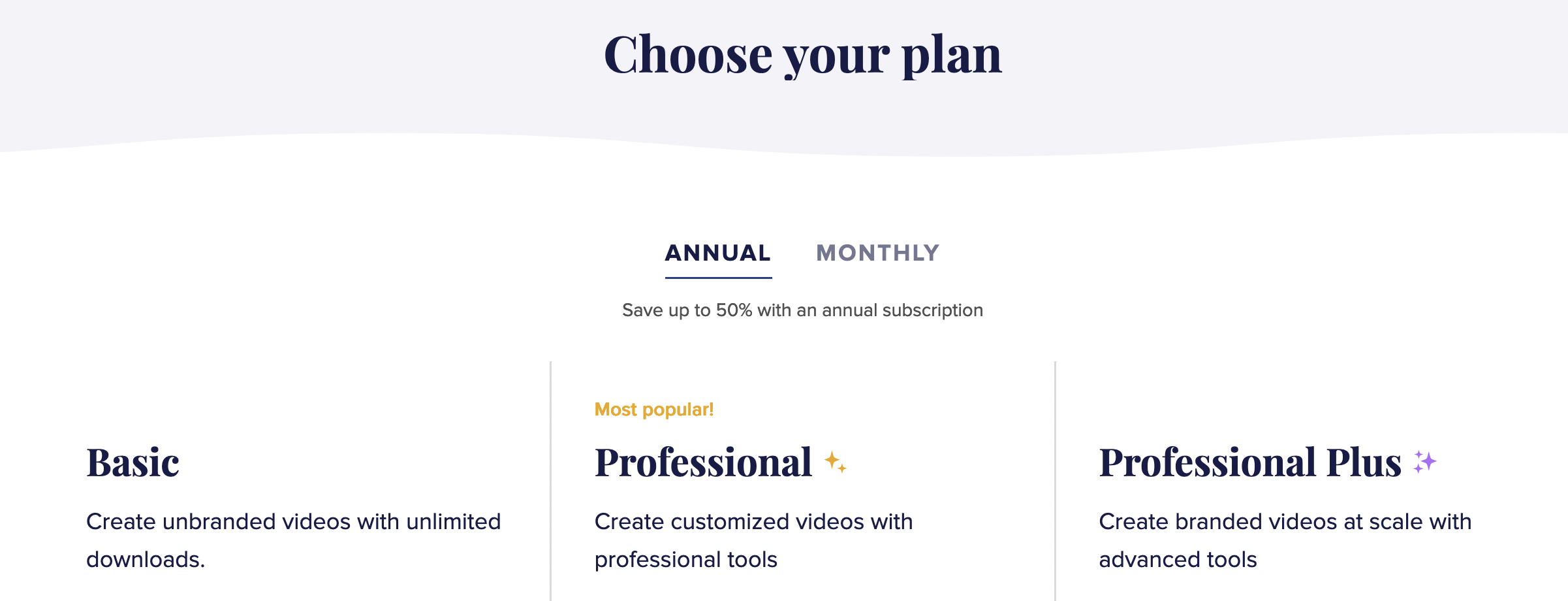The image is a detailed comparison of subscription plans. At the top, there's a heading that reads, "Choose Your Plan." The options are divided into two billing cycles: annual and monthly, with a note stating, "Save up to 50% with an annual subscription."

The plans are categorized as follows:

1. **Basic:** This tier allows you to create unbranded videos with unlimited downloads.
2. **Gold:** Labelled as the "Most Popular," this plan offers the ability to create customized videos using professional tools.
3. **Professional Plus:** The top tier, this plan is designed for creating branded videos at scale with advanced tools, marked by silver or grey accents.

The overall design is sleek, possibly featuring a grey or water-themed background. The call-to-action likely includes interactive elements like "Swipe" or "Wave" to choose between annual and monthly billing cycles, emphasizing the benefits of an annual subscription for cost savings.